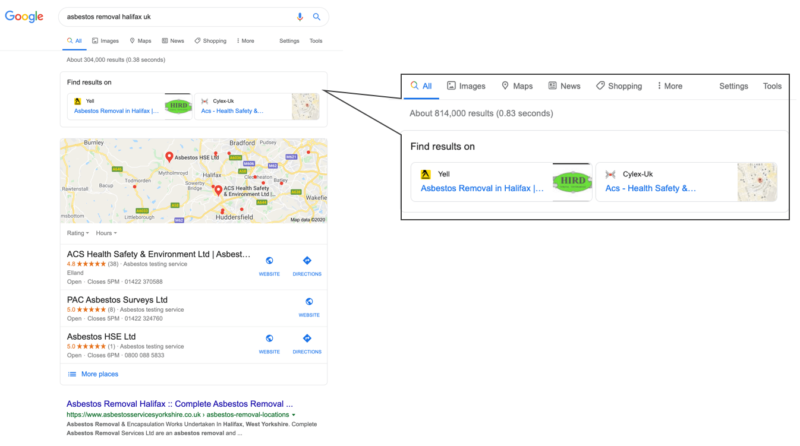The screenshot depicts a Google search results page for "asbestos removal Halifax UK." The search query has yielded approximately 309,000 results in 0.38 seconds. The interface includes standard navigation options such as "All," "Images," "Maps," "News," "Shopping," "More," "Settings," and "Tools." Prominently displayed are Google Maps with a few highlighted businesses offering asbestos removal services in Halifax. 

One listed business is ACS Healthy Safety Equipment LTD, rated 4.8 stars, which provides asbestos removal services. Another option is Pack Asbestos Surveys LTD, which has garnered 5 stars from 8 reviews and offers asbestos testing services, with its operating hours listed until 5 p.m. A third mention includes Asbestos HHE, specializing in asbestos testing services.

The search results provide options such as visiting their websites or obtaining directions directly from the Google Maps interface. At the bottom of the page, there is a section for "Complete Asbestos Removal Halifax" suggesting comprehensive asbestos removal services. The features available for further search refinement include "Find more results in magnify" and resources from "Yell" or "Silent UK". Overall, the Google search effectively provides a variety of avenues for asbestos removal and related services in Halifax, UK.